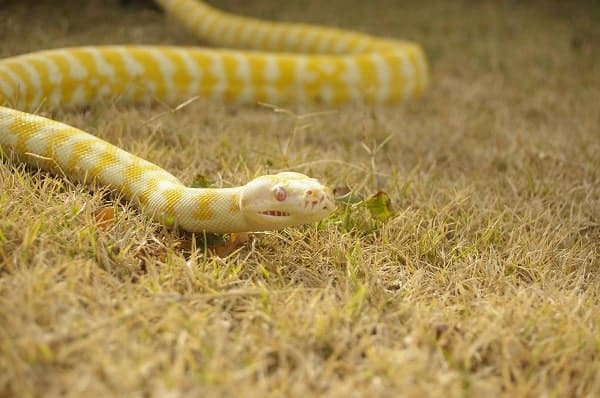This image depicts a striking snake in a sparse and mostly dead grass setting, with some scattered patches of green. The snake's head, which is prominently placed in the middle of the photo, features a curious white coloration with subtle small marks on the right side and an eye that exhibits a yellow-brown hue. The head appears slightly larger, with an intriguing honeycomb-like nose and a partially open mouth showing some teeth. The snake displays a unique color pattern of bright white with light creamy yellow markings. The body, forming a soft 'S' shape, slithers to the left and curves up, disappearing off the upper left edge of the image before reappearing and curling back to the right, and then off the image again. The background, composed of short, thin, brownish grass with sparse green spots, becomes slightly blurry away from the snake's focused head and upper body, emphasizing the snake's prominent position in the scene.